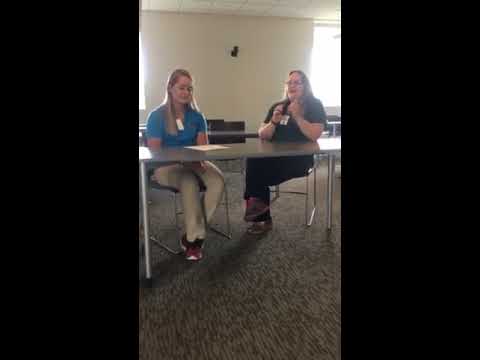The photograph captures two women seated at a table in what appears to be either a conference room or a classroom. They are sitting on plain metal and plastic chairs with visible legs, suggesting the table has no bottom panel. The carpet underneath them is a dark, patterned industrial style typical of institutional settings.

The woman on the left is Caucasian, with long, straight blonde hair. She wears a blue polo shirt paired with khaki pants and red and white sneakers. Her hands are folded under the table as she looks downward towards a paper in front of her. A name badge is fastened to her right.

To her right sits an older Caucasian woman, likely in her 40s, with long dark hair. She is dressed in a black outfit accompanied by brownish shoes and glasses. This woman is angled towards her companion, appearing to be mid-sentence. Both women sport name tags, indicating they might be attending a conference.

The background features an off-white wall and a window on the right side, allowing daylight to stream in, suggesting it is daytime. The image is bordered by black bars on the left and right, focusing the viewer’s attention on the interaction between the two women at the table.